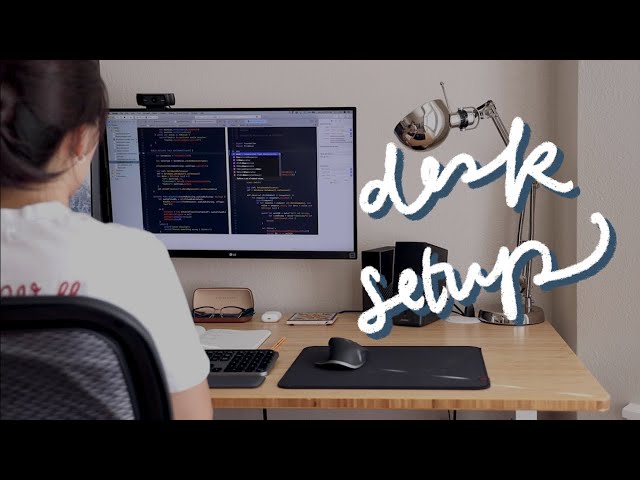This indoor photograph prominently features a meticulous desk setup with multiple items carefully arranged. At the center of the image is a wooden desk, dominated by a black mouse pad with an LED wireless mouse resting on it. To the left of the mouse pad lies a keyboard, directly below an open book and a glasses case containing a pair of glasses. To the right of this arrangement, there is an AirPods case, and nearby, a charging tablet. Further right still, a pair of speakers is visible, all leading up to a sleek, large, silver desk lamp.

Higher up and slightly to the left of the desk, a computer monitor displaying coding information captures the eye, topped with a black webcam. Framing the left side of the image, a woman with brown hands, dressed in a white short-sleeved t-shirt, is seated in a black office chair, evidently engrossed in her work at the computer. Her light-colored skin suggests she may be Caucasian.

Overlaying the right side of the image is white cursive text that reads "desk setup," framed by black borders on both the top and bottom of the photograph, adding a touch of stylistic framing to the overall composition.